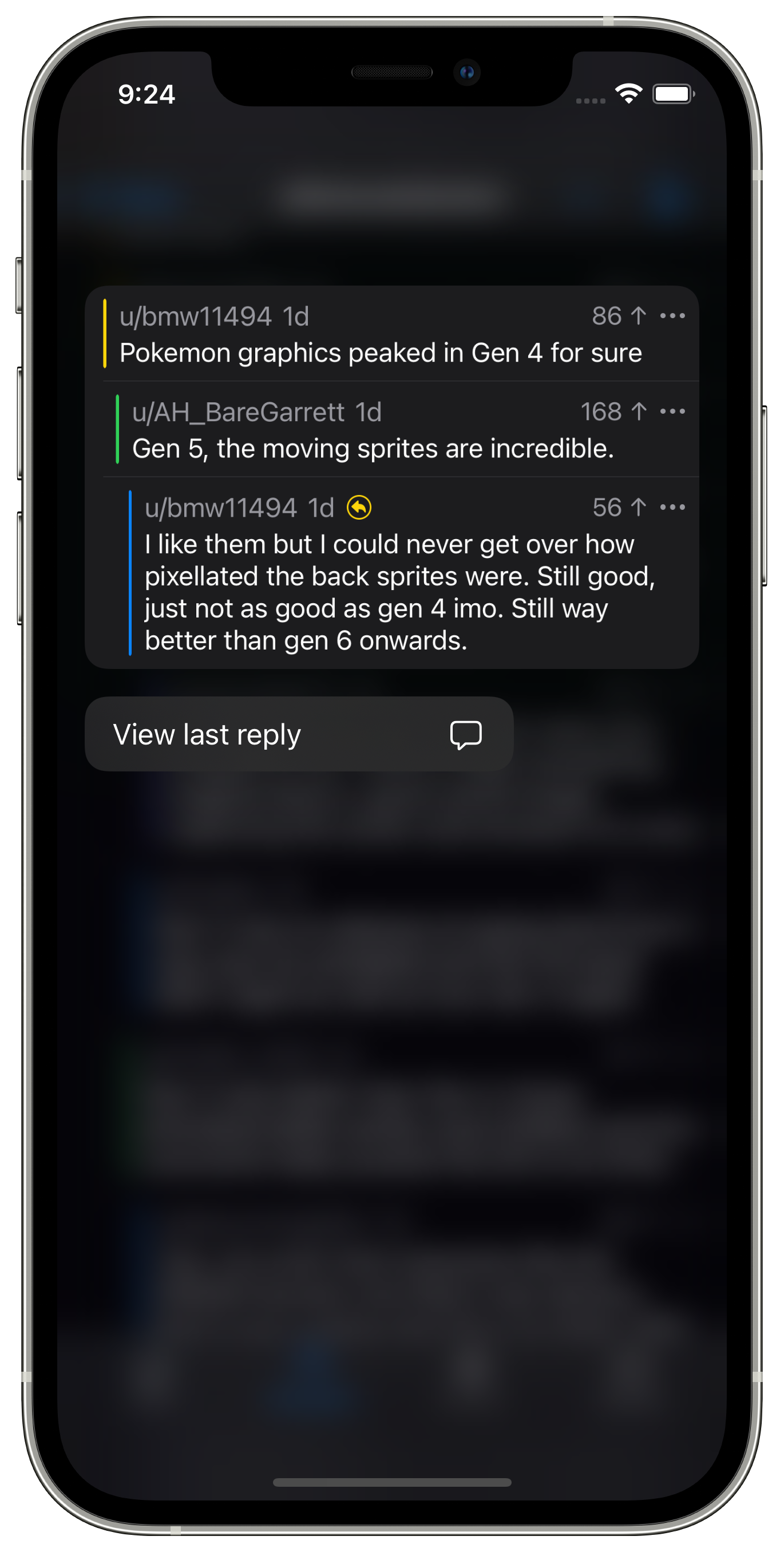In the image, a smartphone screen is displayed prominently. The top left corner of the screen shows the time as 9:24. The phone has no cellular service but full Wi-Fi connectivity, and the battery icon indicates a full charge. The screen is displaying a Reddit thread.

The top post in the thread is from user u/bmw11494, posted a day ago, and has 86 upvotes. The content of the post reads: "Pokemon graphics peaked in Gen 4 for sure." Below this, a reply from user u/ah_bear_garret states, "Gen 5. The moving sprites are incredible." Another reply from u/bmw11494 follows, saying, "I like them but I can never get over how pixelated the back sprites were. Still good, just not as good as Gen 4 IMO. Still way better than Gen 6 onwards." 

Below these comments, there is a small rectangle with a message icon that reads "View Last Reply." The comments are visually emphasized with a 3D effect, making them stand out from the rest of the background, which is a blurred continuation of the Reddit thread.